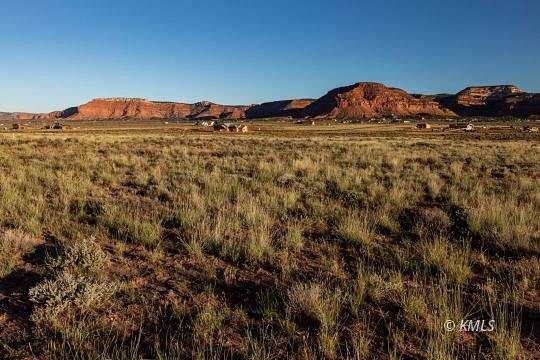In this landscape-oriented photograph captured during the daytime, we see a vast expanse of grassy plains stretching across the foreground. In the distance, a small plateau rises modestly—approximately 20 to 30 feet above the surrounding terrain. The plateau is positioned centrally within the frame and serves as a focal point against the otherwise flat landscape. Midway into the scene, a group of indistinct animals—possibly cattle or buffalo—can be observed grazing. Their forms are somewhat blurred due to their distance from the camera. The sun, positioned to the right, casts shadows that extend gently toward the left, indicating late afternoon light. The lower right corner of the image bears the notation "© KMLS."